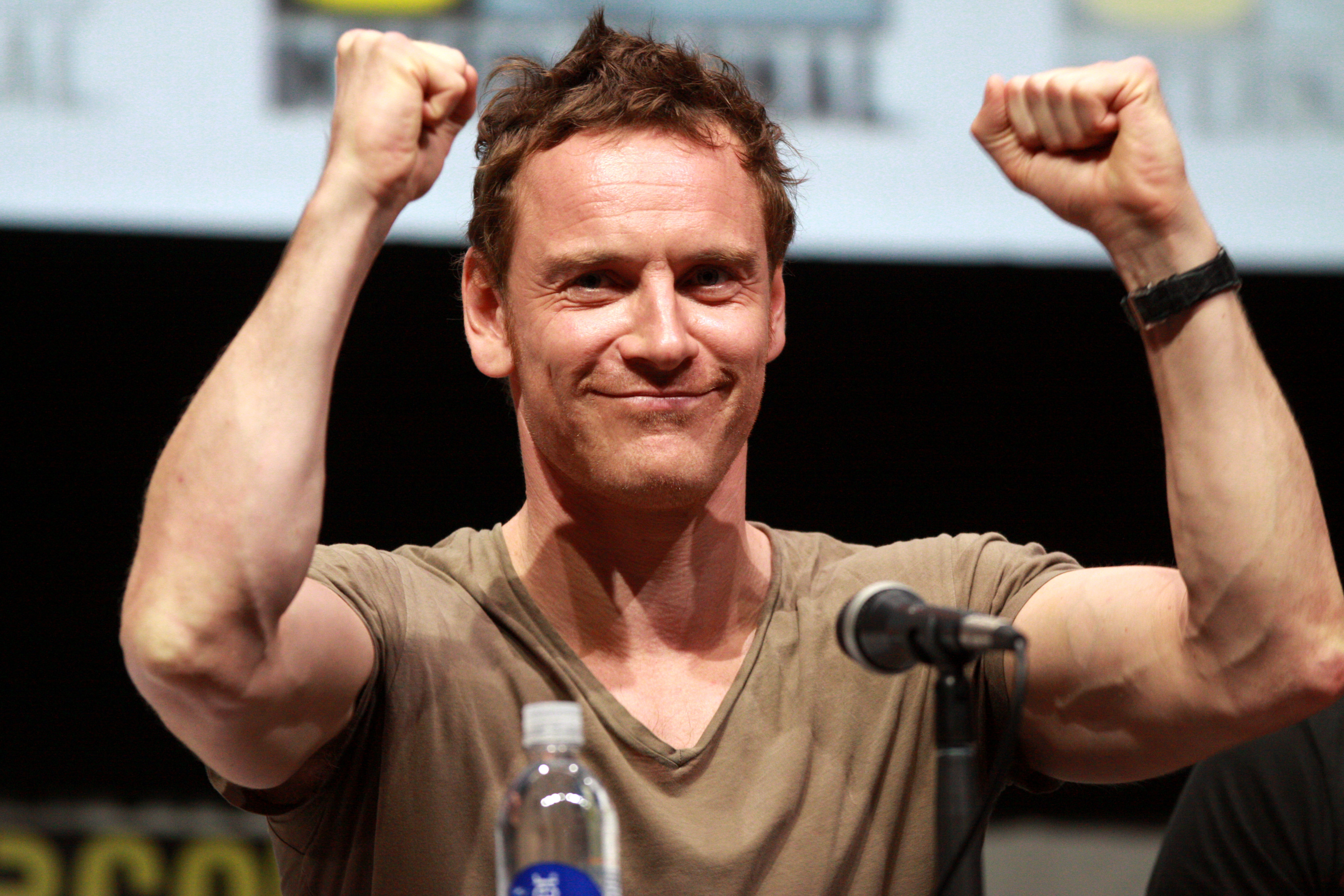In this remarkably detailed image, a muscular man with short, messy brown hair is captured in a moment of triumph and enthusiasm. With clenched fists raised in a victory pose, he's grinning broadly, exuding happiness. He is wearing a light brown v-neck shirt and appears to be standing behind a podium. In front of him on the podium is a black microphone and a bottle of water with a blue logo and a white cap.

To the left of the image, partially blurred yellow digits can be seen. The backdrop behind the man features a white screen or poster with an indistinct logo or text, adding a professional or formal ambiance to the setting. You can discern part of another person seated to the right of the man, indicated by a glimpse of their black shirt. The lighting suggests the photo was taken indoors, as it highlights the man's features clearly, and he seems to be looking slightly off to the right, directly engaging with the moment.